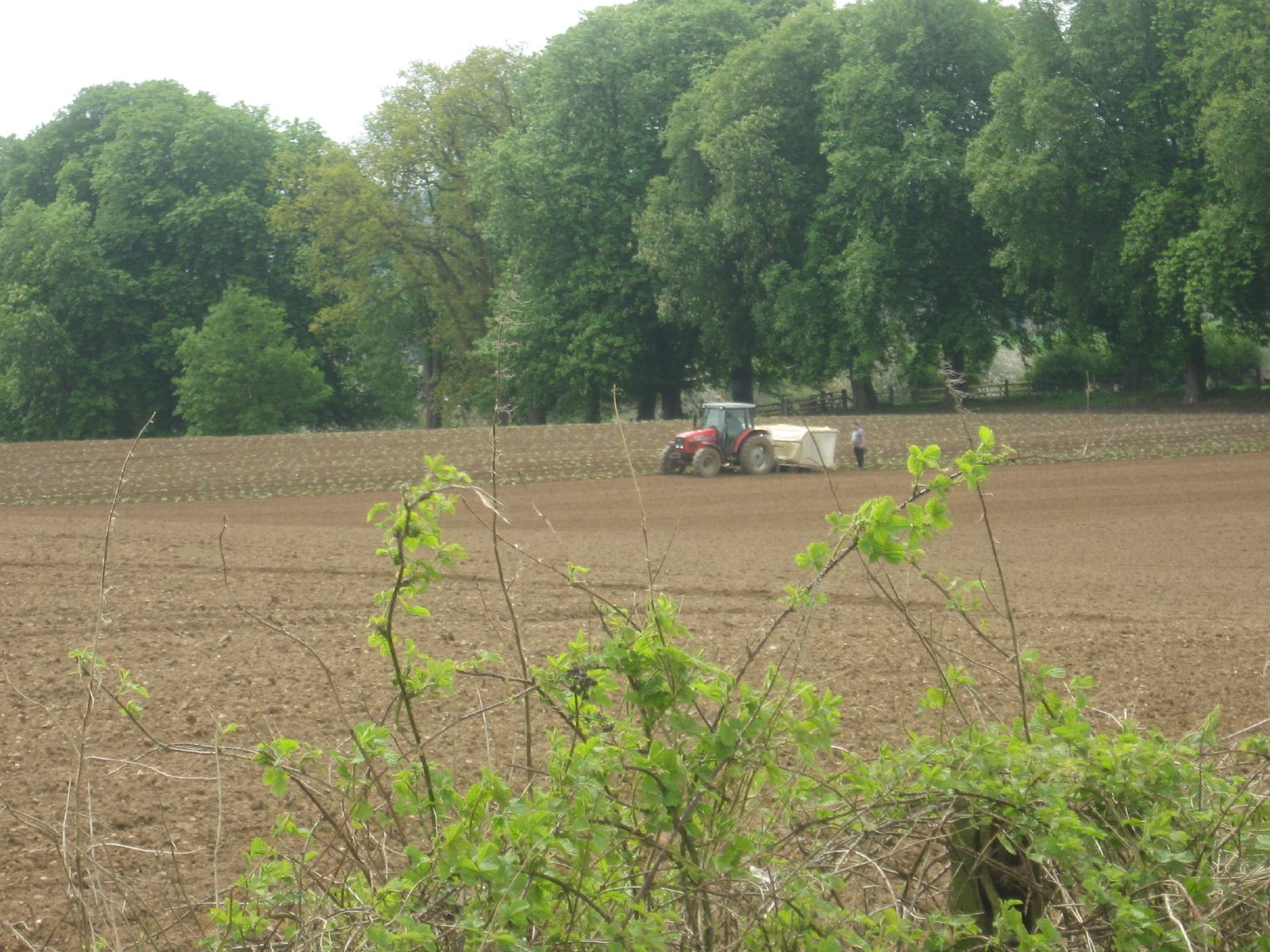In this image, a red tractor is positioned centrally but in the distance, giving it a smaller appearance against the vast expanse of a large farm field. The tractor appears to be involved in planting activities, as evidenced by half of the field already being planted. The rest of the field remains untouched, and the tractor seems poised to continue its work. The earth in the farm field is mostly bare, except where planting has occurred. A man stands behind the tractor, examining a white box attached to it, which is likely part of the planting equipment.

The backdrop features towering, lush green trees, enclosed by a small wooden fence. In the foreground, green shrubs, vines, or plants are also visible, suggesting that the photograph was taken during the summer. The entire scene depicts a quintessential summer day on a farm, with an emphasis on agricultural activity framed by verdant foliage.